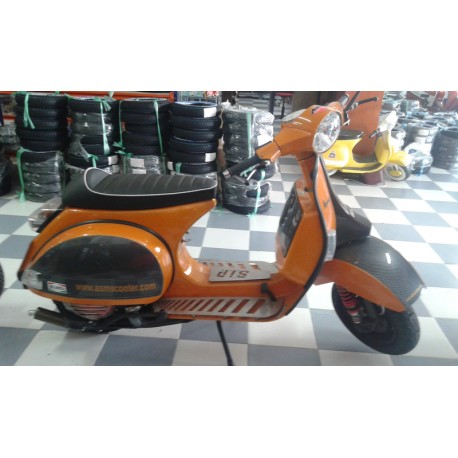In this image, we see a detailed and vibrant setting, likely inside a motorcycle shop, captured in the middle of the day under bright indoor lighting. Dominating the scene is a prominently centered orange motor scooter, painted in a distinctive Harley Davidson shade. The floor beneath the scooter is a black-and-white checkered linoleum, giving the impression of a showroom display.

The scooter features a black seat outlined with a thin white border, and its body carries a black or possibly gray racing stripe down the front. The handlebars are tilted to the lower half of the image, and they end in black rubber grips. A capsule-shaped white headlight is positioned at the front, contributing to its sleek appearance. The scooter stands on a black kickstand, giving it stability on the floor.

The scooter's rear fender displays a website address, www.scooter.com, while its wheels are solid black, with the rear wheel well encased in black bordered by orange. Notably, the spokes of the front wheel bear the letters STP. 

In the background peeking out are stacks of tires and another scooter, indicating that the setting is likely a busy and well-stocked motorcycle shop. The array of colors in the image includes gray, white, orange, black, green, yellow, and silver, which adds vibrancy and detail to the composition.